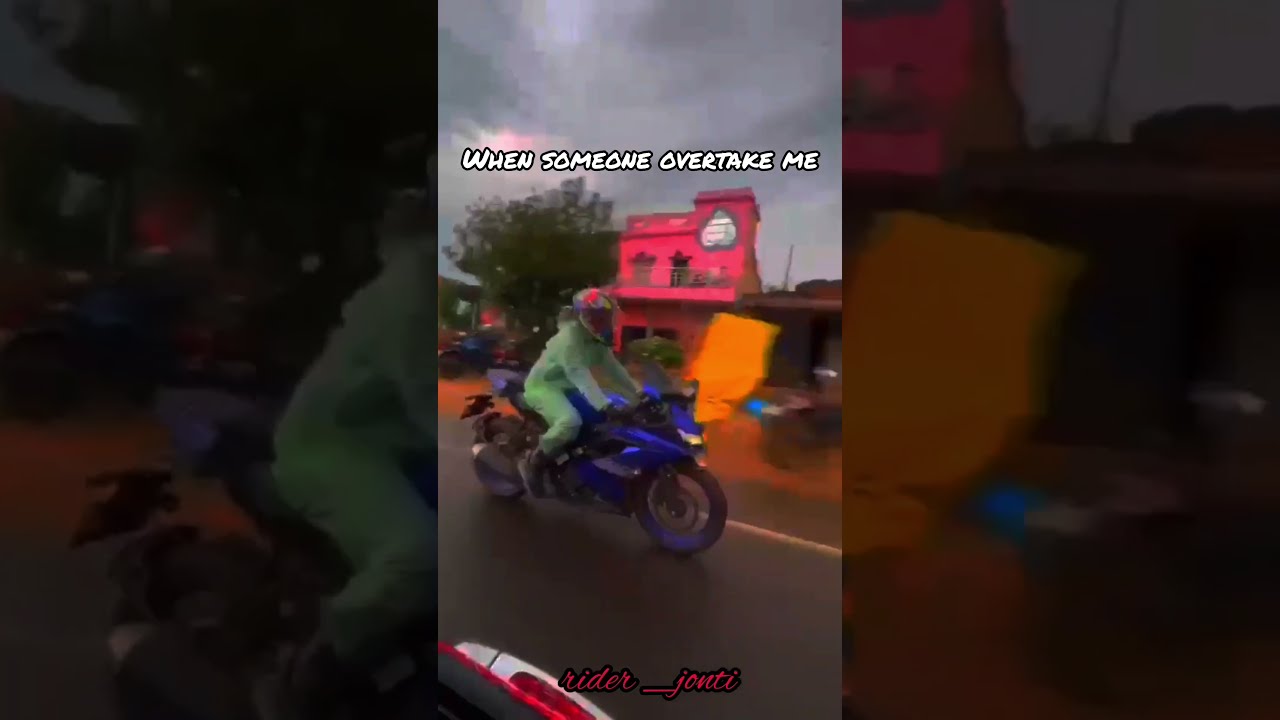The image displays a daytime outdoor scene, characterized by a gray, overcast sky with numerous clouds. Central to the image is a man riding a blue motorcycle on an asphalt road marked with a white stripe. The rider, in a light green long-sleeve outfit, matching pants, and boots, dons a helmet adorned with pink and white streaks. The backdrop features several trees and buildings, including a prominent two-story pink house and another orange-colored structure, hinting at a more urban setting. The image has textual overlays: "When someone overtake me" in small, white letters with black outlines at the top center, and "rider_jaunty" in cursive pink font with a black outline at the bottom. The scene has a slightly dark, foggy ambience, yet remains clear enough to convey the details, suggesting the image was taken on a less sunny day. The picture appears to be part of a meme intended for social media, emphasizing humor and relatability for riders.